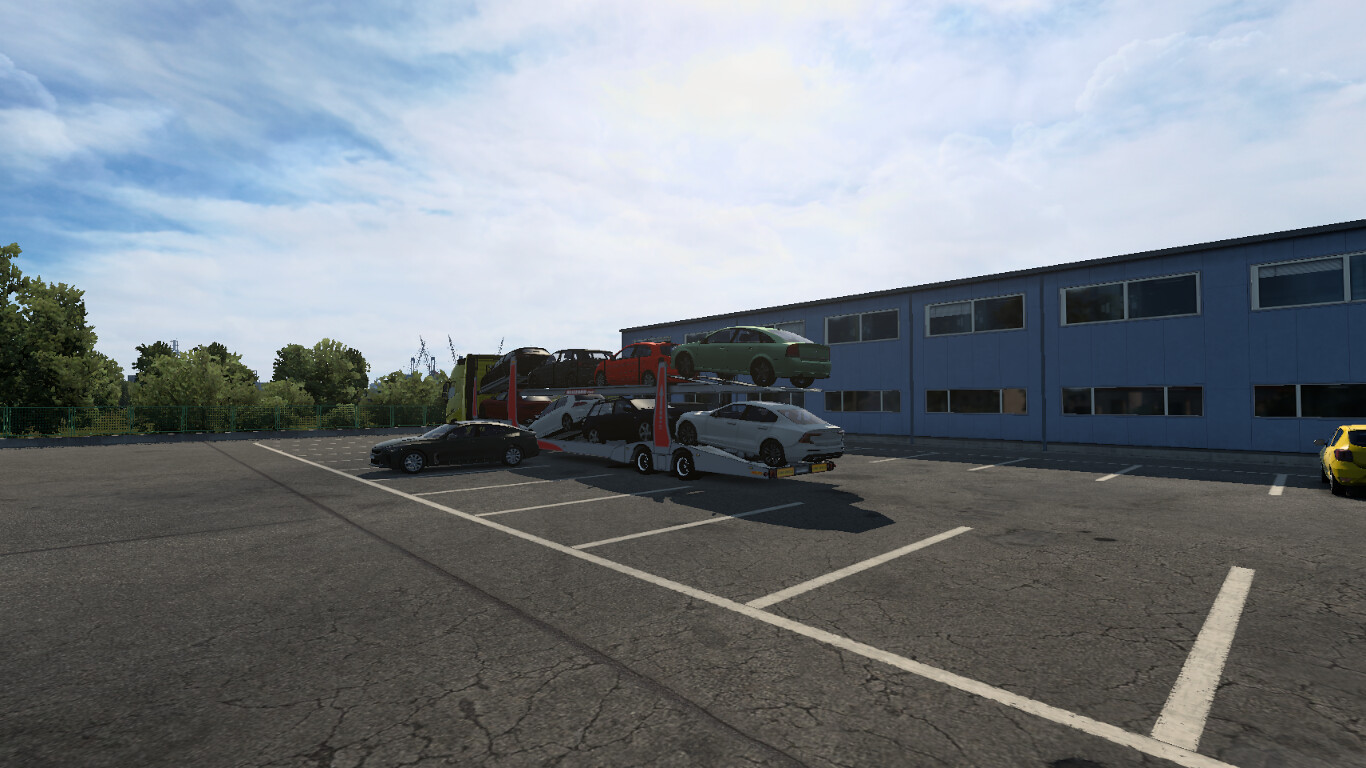In an expansive, cracked asphalt parking lot with clearly painted spaces, a yellow-front car carrier holds eight Chrysler vehicles, including a Dodge Charger. The lot is mostly empty except for a few other cars—a yellow and a black car. Dominating the backdrop is a plain, two-story blue building, suggesting a motel or similar lodging. The structure is unremarkable, with uniformly repetitive windows that differ between the two stories. Large, lush green trees and an overcast, cloud-filled sky frame the scene, while shadows from the vehicles and objects add depth to the otherwise tranquil setting.